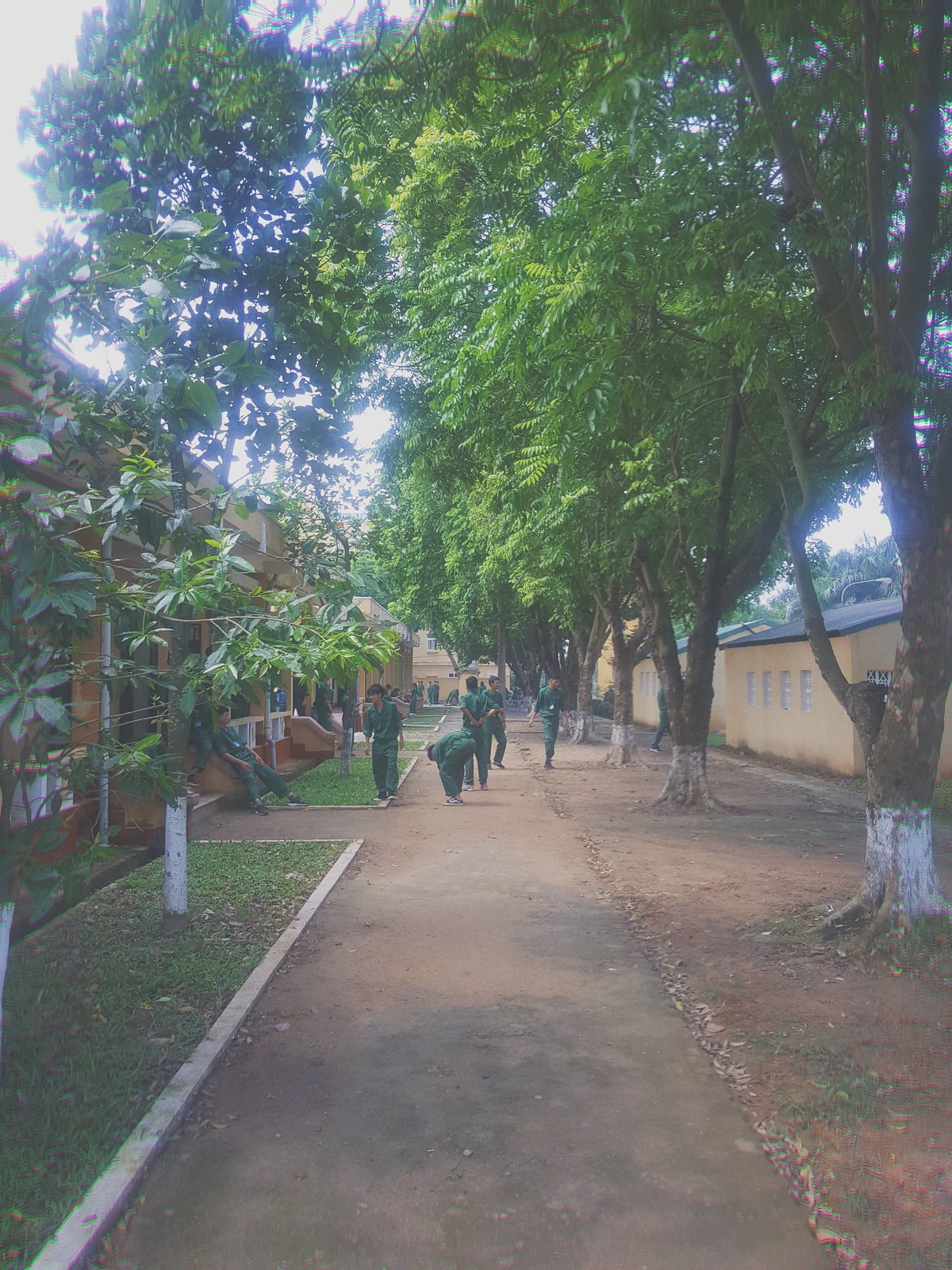The photo captures an outdoor scene featuring a well-maintained walkway flanked by various landscape elements and buildings. To the left of the path, there are patches of grass bordered by white stone, while the right side is lined with small stones creating a border around a mostly dirt area from which trees grow. The trees, which have their bases painted white, provide a canopy of lush green leaves that offer some shade over the walkway. 

In the background, there are several individuals who appear to be men or boys, all dressed in dark green outfits comprising long-sleeved shirts—some with sleeves rolled up to the elbows—and long pants. These individuals are uniformly attired, but the outfits do not resemble military uniforms and instead give an impression of prisoner garb or some form of institutional clothing. Some of them wear white badges around their necks, adding to the sense of uniformity.

The pathway, made of dirt, stretches into the distance and is lined with buildings on both sides. The structures on the left are in a yellow stucco finish with dark roofs, and some individuals can be seen lounging on the steps of these buildings. The right side remains more earth-toned, emphasizing the dirt beneath the trees. White light filters in from the top left corner, casting a subtle illumination over the somewhat muted and dull atmosphere of the scene.